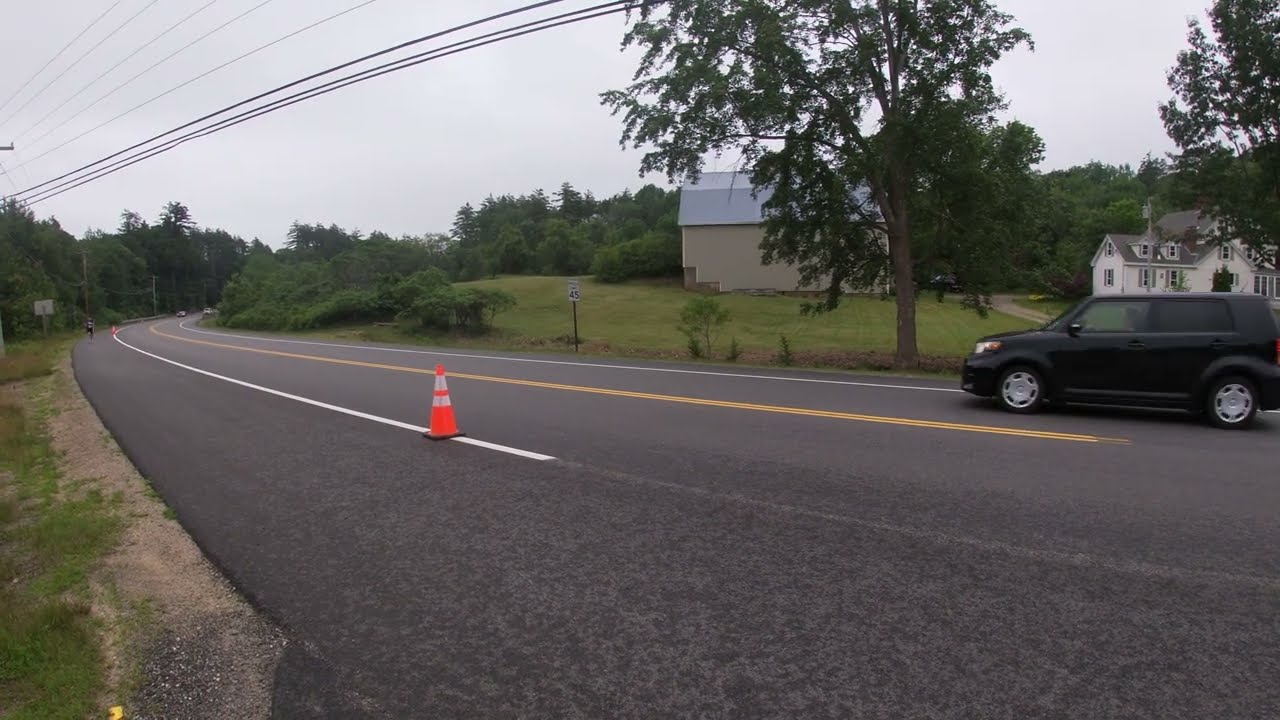The image depicts a country road with a two-lane blacktop featuring a double yellow line down the middle. The road curves off to the right before disappearing out of view. A black SUV, potentially a Kia, is driving from right to left on the right lane, adjacent to the double yellow line. The road appears freshly paved and has white bike lanes on either side marked by several orange traffic cones. Farther down the road on the shoulder, a person is visible, possibly signaling a road race or another event. Power lines, slightly curved due to a fisheye effect, run across the scene from above. On the right side of the image, there's a large white barn and a house, both surrounded by green fields. Trees and vegetation line the sides of the road, and the sky is cloudy, adding a somber hue to the overall daytime setting.